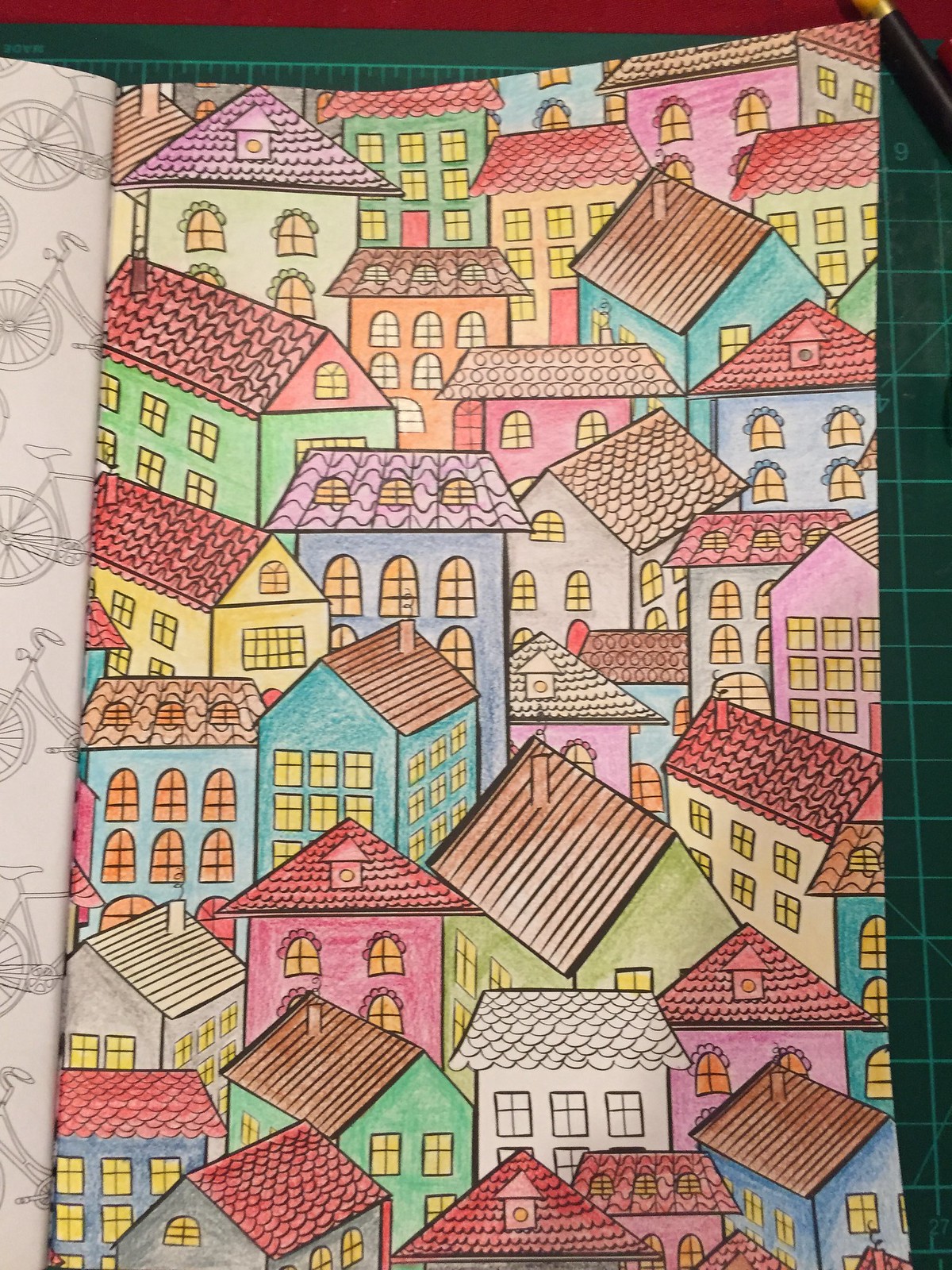This drawing appears to be inspired by a quaint cityscape, reminiscent of an old-fashioned greeting card. The artwork features an assemblage of houses closely packed together, creating an intricate, almost chaotic, yet charming urban cluster. The houses are oriented in various directions rather than neatly aligned, giving the scene an organic, lived-in feel.

Each house is topped with a peaked roof, varying in color. Predominantly, the roofs are brown or red, with a few notable exceptions, such as a couple of purple roofs and a solitary gray one. Many of these homes are adorned with numerous windows, some of which glow with a warm yellow light, suggesting that they are inhabited. Others present a more subdued appearance with dark brown windows.

The main scene is centered, but the left side of the image reveals another page, perhaps from a book, which is illustrated in black and white featuring bicycles. At the top of the image, there is a splash of green and red, adding a vibrant touch. More green hues are found on the right side, framing the densely packed houses and adding to the overall sense of whimsy and charm in the drawing.